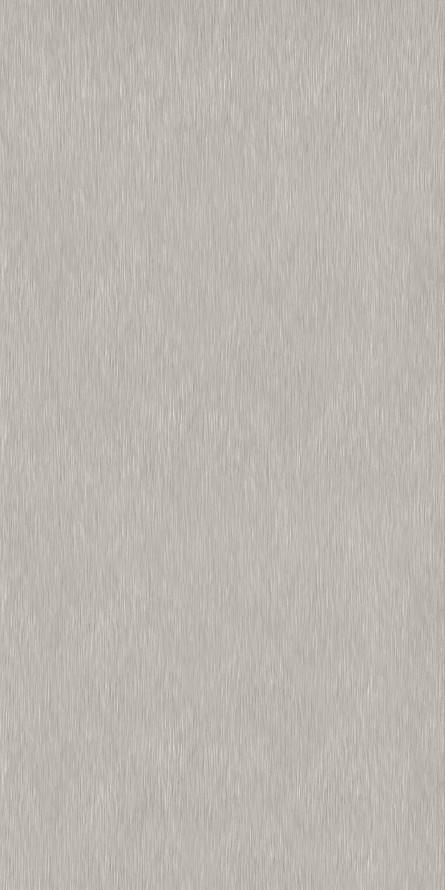The image depicts a tall, vertical, rectangular piece that appears to be a sample of vinyl flooring. The plank has an elongated, narrow shape, approximately three times longer than it is wide, with a height of about three inches and a width of around one and a half inches. The color palette transitions from a darker gray at the top to a pale gray and beige towards the bottom, interspersed with subtle white speckles and striations that create a faintly textured, organic pattern. This texture runs vertically, forming an irregular, yet cohesive design. There are no distinguishable objects or text within the image, which is centrally placed slightly to the left on the page, leaving the focus solely on the flooring sample's subtle intricacies and color variations.